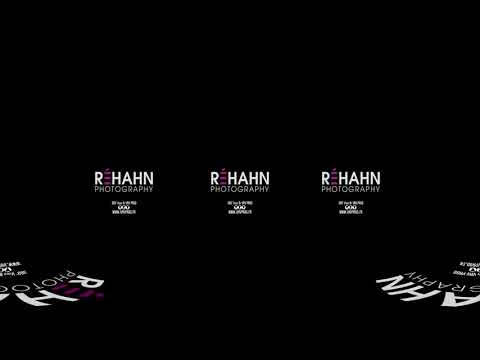The image is a screenshot of a photographer's website featuring the logo "R. Hahn Photography" displayed prominently three times across the center of the screen in bold white text. Each repetition of the logo includes "PHOTOGRAPHY" in thinner gray letters underneath, accompanied by three horizontal red lines with a red circle above between the "R" and "H". The background is black, providing a stark contrast to the bright text. Additionally, the logo appears partially and upside down in the bottom left and right corners of the image, with the left side showing "R" and "H," and the right side showing "A H N" and "P H O T O" (cut off). The text beneath the logos is too small and blurry to be legible. The sophisticated and symmetrical layout emphasizes the photographer's brand, creating a striking visual effect.